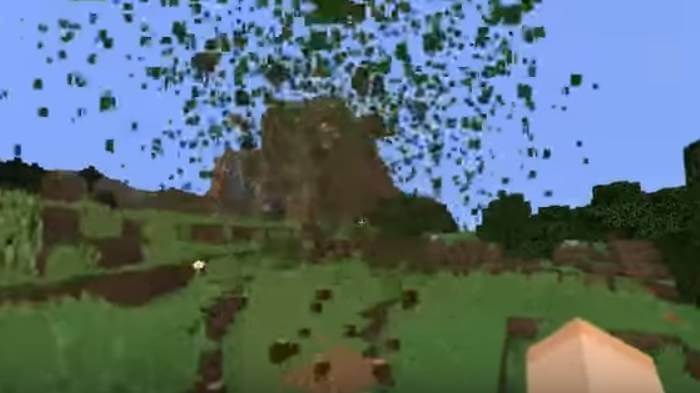This screenshot from an old video game showcases a highly pixelated, retro aesthetic with basic graphics. The upper portion of the image features a sky shaded in a simple blue, devoid of intricate details. Dominating the center is a massive rock formation or mountain, providing the main visual focus. Surrounding this rock are numerous green, geometrically-shaped pixel chunks that appear to be flying through the air. These green blocks are densely clumped near the rock but become increasingly sparse as they disperse further away.

On either side of the rock formation, patches of green vegetation are visible, adding some color contrast to the scene. Below the vegetation, there's an additional rocky barrier that wraps around, creating a layered terrain. In the bottom right corner of the screenshot, a rectangular or square object protrudes into the frame, its purpose unexplained but contributing to the overall vintage game environment.